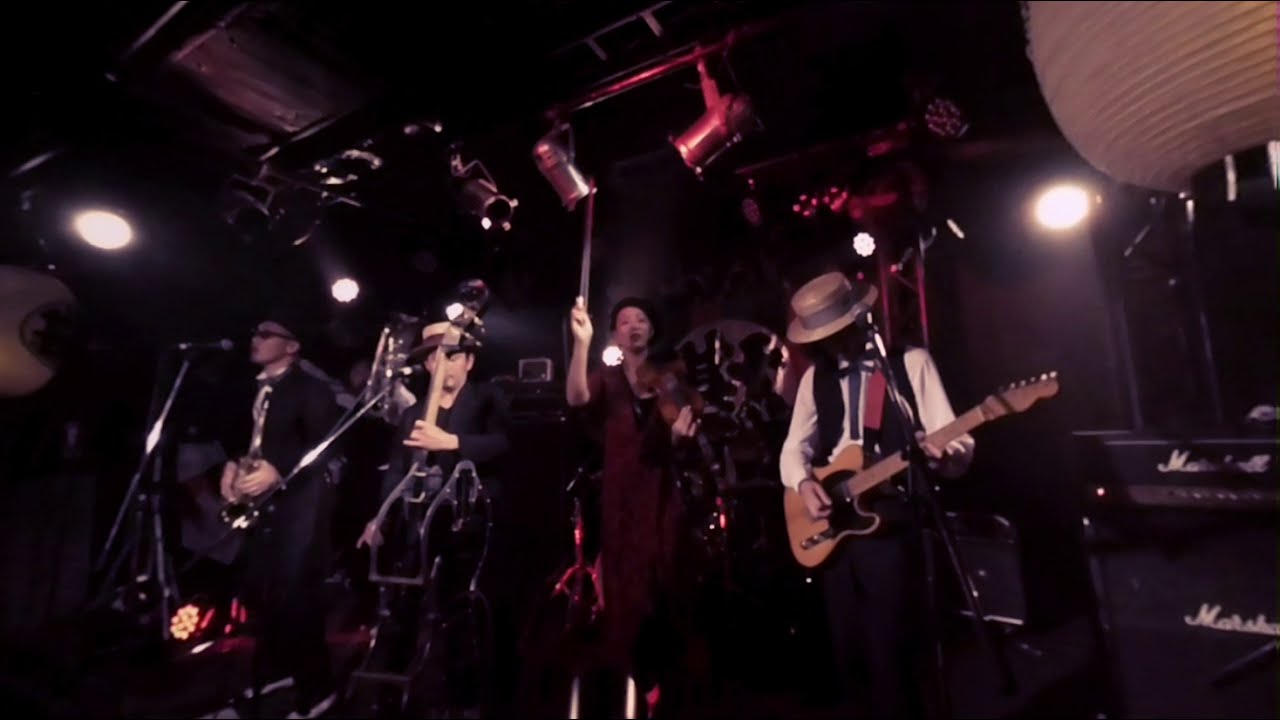The image captures a blues band in mid-performance on a dimly lit stage, reminiscent of a small club setting. Four musicians are present, each contributing their unique style to the ensemble. On the far right, a male guitarist is seen wearing a broad-brimmed straw hat, a black vest, black pants, a white button-up shirt, and a necktie. His head is bowed as he skillfully plays the guitar. To his left, a woman dressed in a striking dark red dress holds a violin in one hand and raises the bow with the other, her hair pulled back neatly. The third musician, positioned further left, plays an upright bass that appears to be made of a transparent material, possibly plastic or resin. He also sports a broad-brimmed hat. On the far left stands a man dressed in a dark suit, with a white button-up shirt, and black hat. He is singing into a microphone while holding a saxophone, with dark sunglasses accentuating his stage presence. The stage is enveloped in darkness, with only the stage lighting highlighting the performers, creating a somewhat murky but intimate atmosphere.